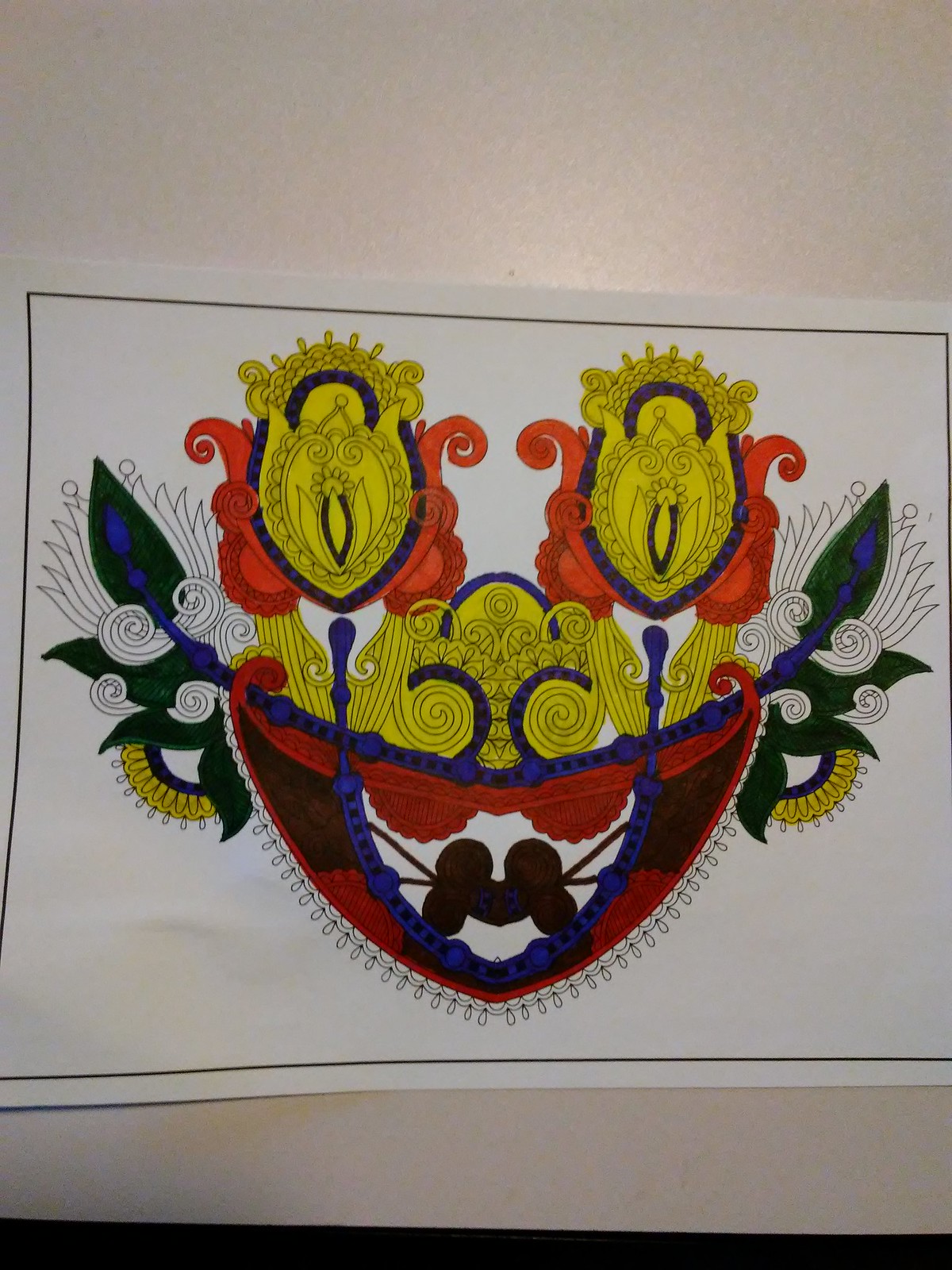The image depicts an intricately designed crest, likely drawn with markers due to its rich, dark colors. The central element resembles a stylized fruit bowl, though with spiral accents rather than actual fruit. The lower section of the crest is predominantly colored in red and maroon, featuring scoop-shaped flags beneath it. The background of the image is white, while the crest itself is rendered in brown, with blue trim framing either side. The top portion of the crest is adorned with numerous lines and circles crafted in gold.

Above the main body of the crest are two tulip-like forms, characterized by red sides and scalloped gold patterns. These tulips are outlined in black and crowned with gold decorations. On either side of the crest, golden handles adorned with green leaves add to the ornate appearance. The entire composition is set against a tan background, enhancing the detailed and vibrant elements of the crest.